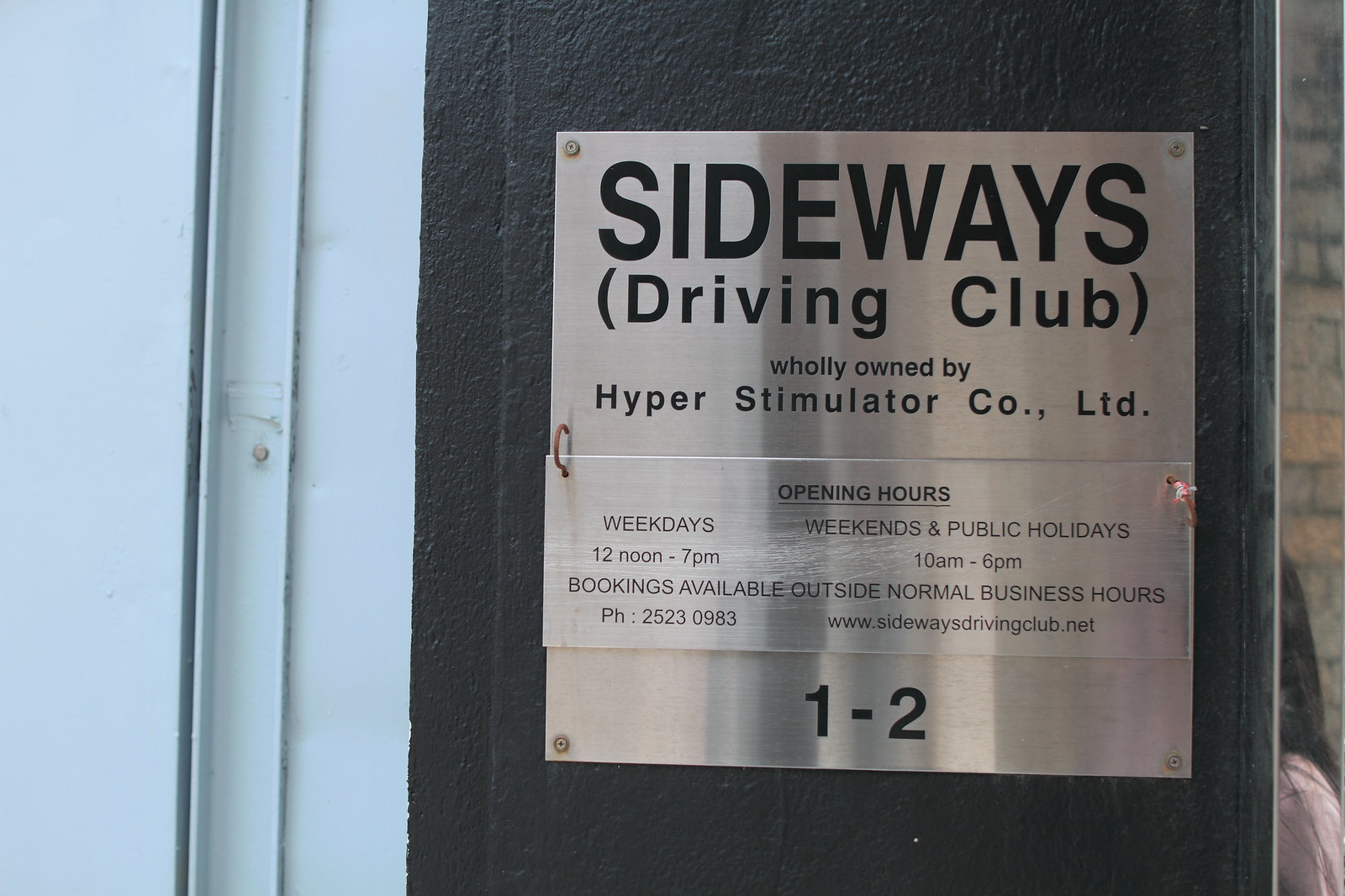The image depicts a stainless steel sign affixed to a black pole situated to the right of a light blue wall. At the top of the sign, "SIDEWAYS" is prominently displayed in black, all-capital letters. Directly below, in parentheses, it reads "Driving Club". Following this, the sign states "Wholly Owned By" and "Hyper Stimulator Co Ltd". At the very bottom, the text "1-2" is visible. Central to the sign, there is a metal plaque detailed with "Opening Hours," listing "Weekdays: 12 noon to 7pm" and "Weekends and Public Holidays: 10am to 6pm". In the background, a barely visible person stands, juxtaposed against a brick wall.